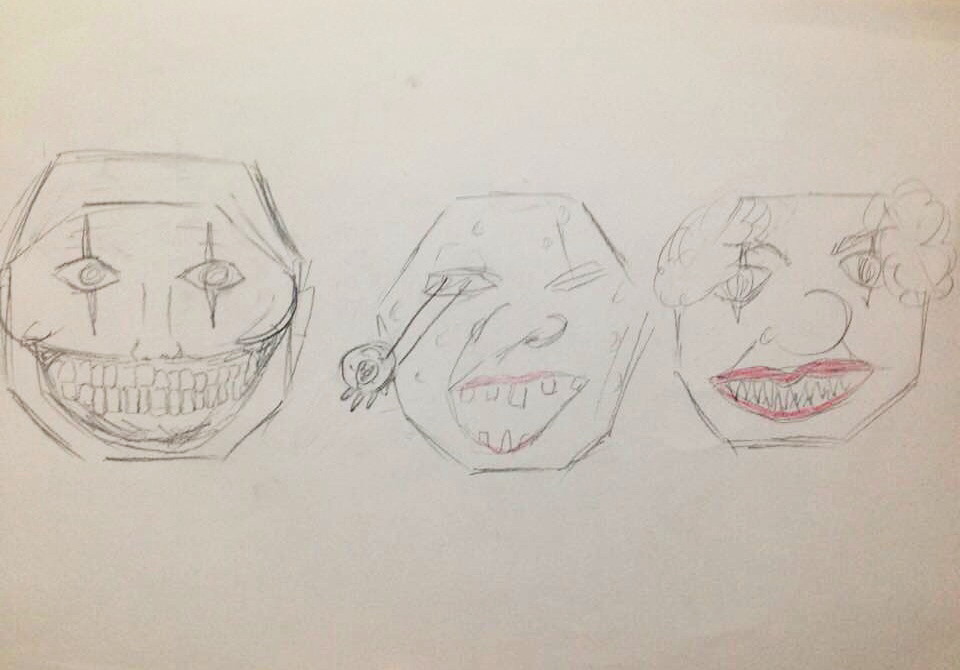This image is a scanned or photographed reproduction of a traditional landscape-style pencil sketch on off-white paper. The composition features three distinct faces, each arranged in a row and possessing an angular, hexagonal—or potentially octagonal—shape. These faces are stylized in a whimsical, clown-like manner reminiscent of gestures or clown figures, possibly inspired by the Insane Clown Posse. The central and right-side faces are accented with red colored pencil around their grinning lips, while the left-side face is rendered solely in graphite pencil. The shading in the drawing adds depth and dimension, suggesting meticulous attention to detail by the artist.